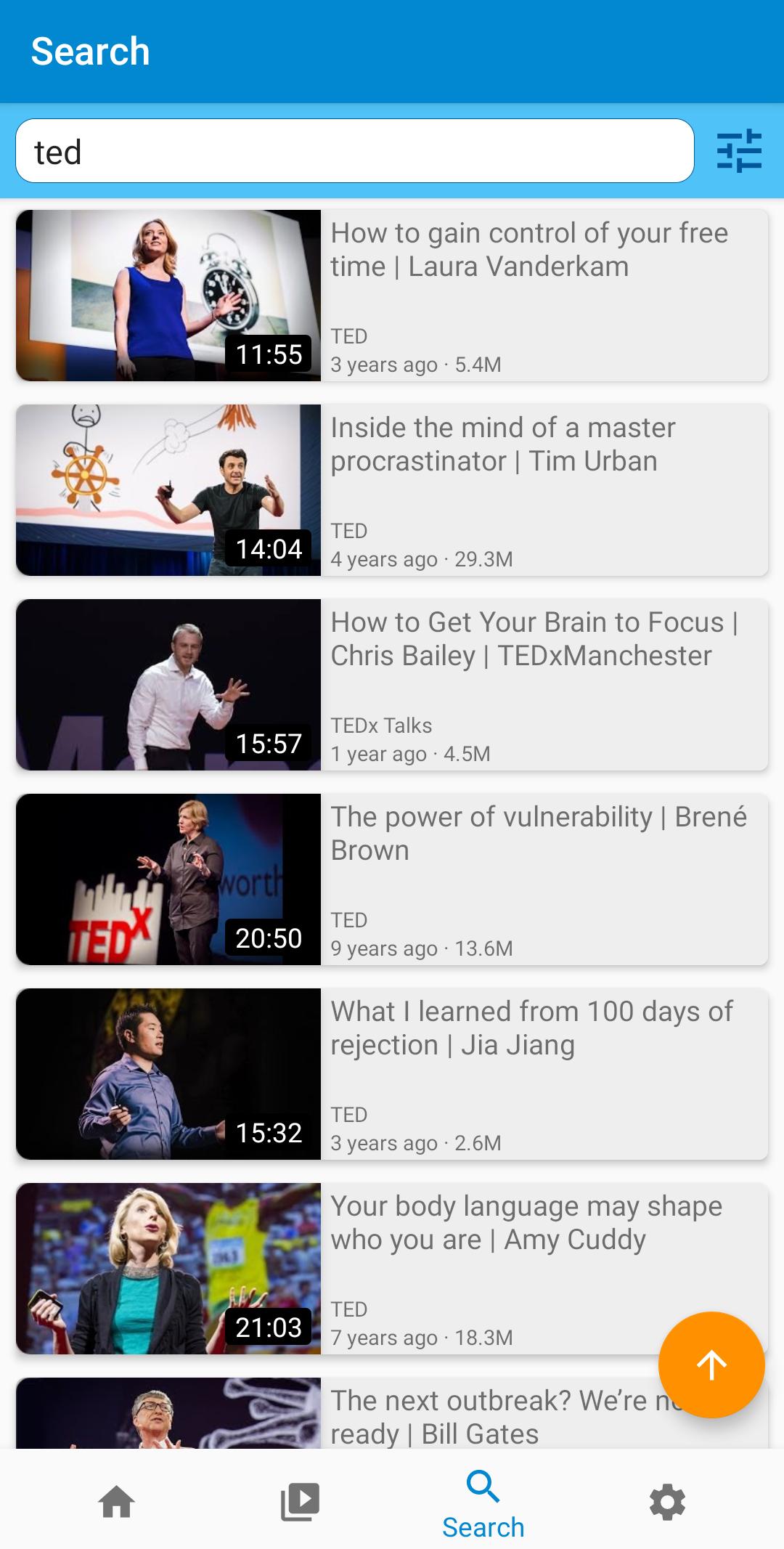The image showcases a selection of notable TED Talk videos available on YouTube, complete with their respective thumbnails, durations, and view counts. At the top of the image, there is a blue banner featuring a white "Search" label. Directly below, a white search bar is set against a sky blue background and is marked with the "TED" logo. A three-bar icon on the left side of the search bar allows users to filter their search results.

The thumbnails and details of various TED Talk videos are listed vertically beneath the search bar. The first video, titled "How to Gain Control of Your Free Time" by Laura Vanderkam, is 11 minutes and 55 seconds long, and shows Laura in a blue shirt standing in front of an alarm clock image. The second video, "Inside the Mind of a Master Procrastinator" by Tim Urban, lasts 14 minutes and 4 seconds. The third video, "How to Get Your Brain to Focus" by Chris Bailey from TEDxManchester, is 15 minutes and 57 seconds long, has been viewed 4.5 million times, and was uploaded one year ago.

The fourth video is "The Power of Vulnerability" by Brené Brown, lasting 20 minutes and 50 seconds, with 13.6 million views from nine years ago. The fifth video, "What I Learned from 100 Days of Rejection" by Jia Jiang, is 15 minutes and 32 seconds long, has garnered 2.6 million views, and was uploaded three years ago. Another video titled "Your Body Language May Shape Who You Are" by Amy Cuddy is 21 minutes and 3 seconds long, has 18.3 million views, and was posted seven years ago. Lastly, there is "The Next Outbreak? We’re Not Ready" by Bill Gates.

Each video description on the left is accompanied by respective thumbnail images of the speakers during their presentations.